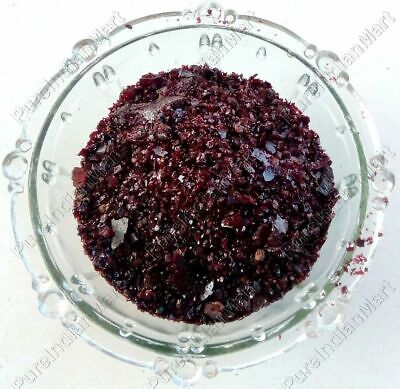This image captures a small, vintage glass bowl with intricate decorations, particularly a textured, non-smooth rim that has small elements protruding. The bowl’s sides steep down vertically from a greenish circular band at the top. Inside the clear but potentially white-hued bowl, there’s a dark, almost black substance, possibly comprised of chopped dates, chocolate chips, or another type of very dark food with a few lighter specks interspersed within. This dark content includes larger flat flakes that may appear grayish, contrasting with smaller, rounded pieces. The image also indicates some spillage on the lower right edge of the bowl, suggesting a lack of a serving utensil. A faint watermark is observed in the background, subtly marking the image. The overall appearance projects a sense of fragility and weight due to the material and contents.